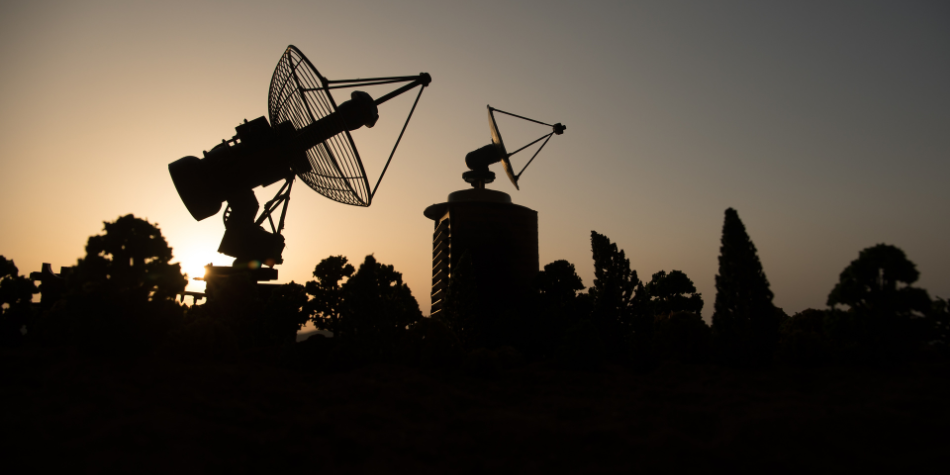This photograph captures the haunting silhouette of two satellite dishes perched on sturdy platforms against the dramatic backdrop of a setting or rising sun. The sun, positioned low in the sky on the left side of the image, casts a hazy, yellow-to-dark-blue gradient across a clear sky, adding an ethereal glow to the scene. The foreground features the darkened silhouettes of various tree species, including both pine and deciduous trees, along with an indistinct small structure or post.

Dominating the scene, the satellite dishes have distinctive forms - one with a metal mesh bowl-shaped receiver supported by a tripod-like structure, and the other with a similar bowl shape leading up to a triangular point. These devices angle upward at approximately 20-30 degrees from horizontal, pointing skyward as if reaching for signals from the cosmos. The juxtaposition of the technological silhouettes against the natural forms of the trees and the serene sky creates a stunning visual symphony, emphasizing the contrast between human innovation and the natural world.